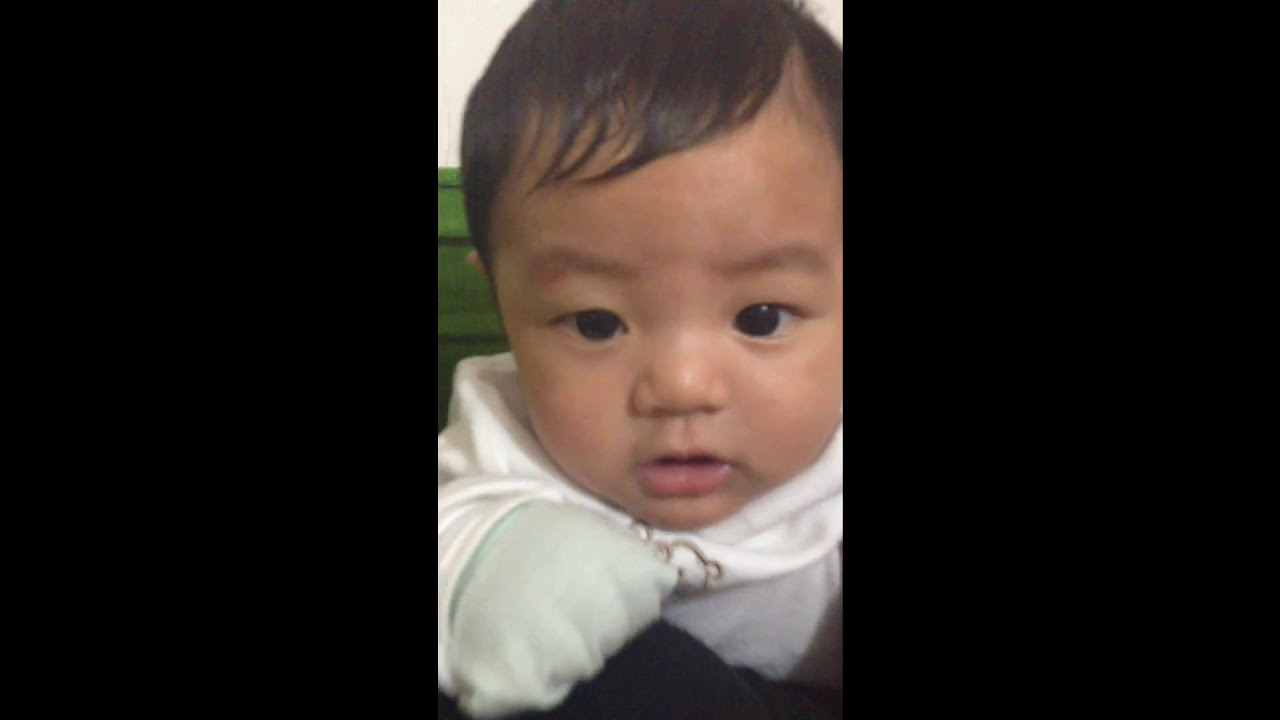This photo is a close-up shot of the head of an infant with very dark hair brushed to the right, featuring a slight wave on the forehead. The baby has dark eyes with a wide, pudgy nose, chubby cheeks, and slightly parted pink lips. The baby is wearing a white top, which appears to be a shirt or hoodie, along with white gloves, with the fingers folded into a fist. The top has an unidentifiable drawing outlined in brown. The baby is positioned on a black material, and in the background is a green area, possibly a cushion or part of a couch, with a white wall above it. The image itself is framed by two large black borders on the left and right, making the overall photo look narrow with no borders at the top or bottom.